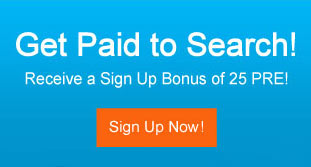The image is a straightforward advertisement for a sign-up program on an unspecified website. The background features a gradient of sky blue, starting lighter at the top and transitioning to a slightly darker shade towards the bottom. Bold white text at the top reads "Get Paid to Search!" with each word capitalized. Beneath this, in slightly thinner white text, the advertisement promises, "Receive a Sign-Up Bonus of 25 PRE!" with the key words also capitalized for emphasis. At the bottom of the image, there's a prominent orange button with capitalized white text that says, "Sign Up Now!"